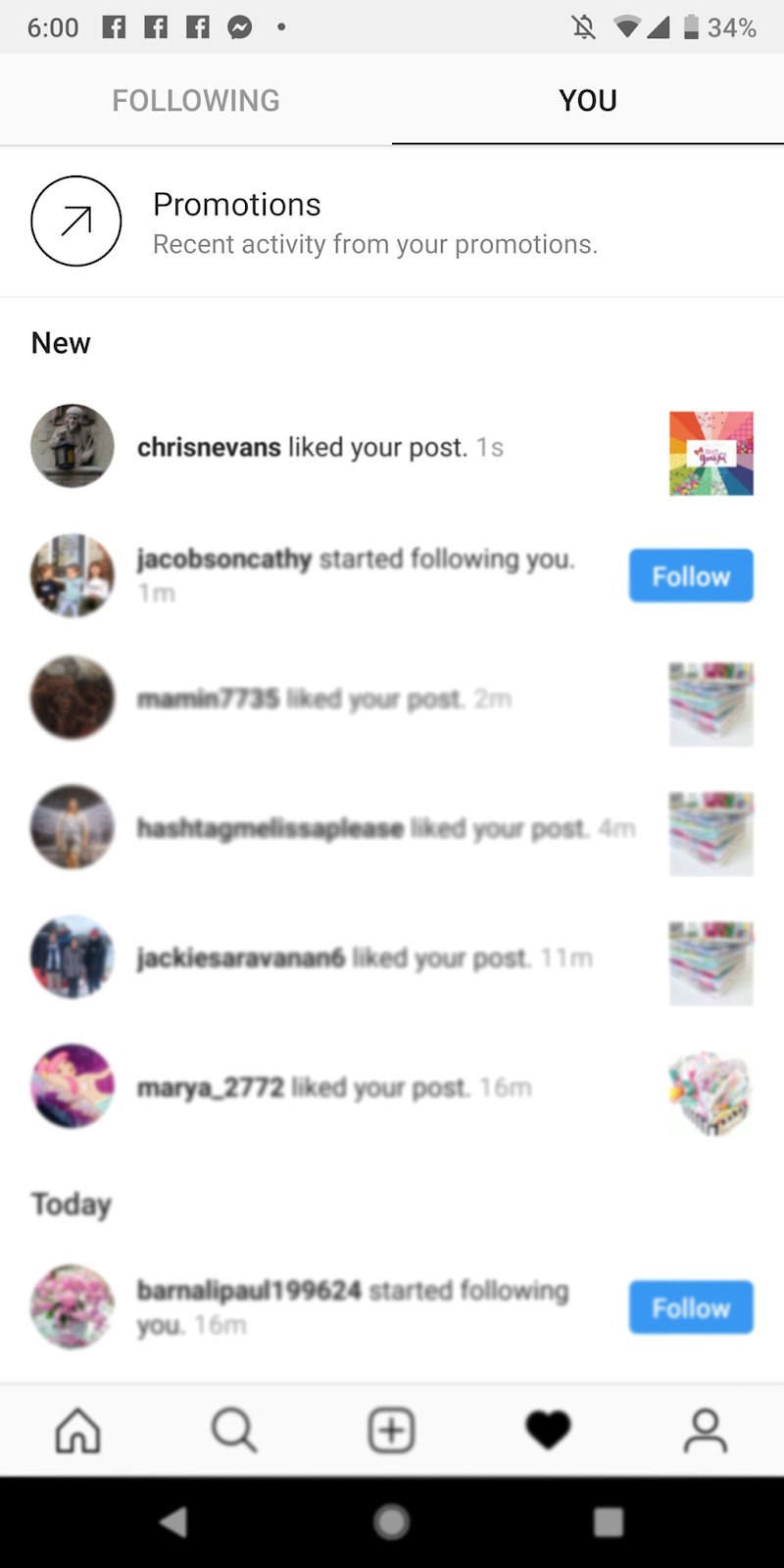The image is a vertically rectangular screenshot from a cell phone. At the top left corner, the time is displayed as 6 o'clock. Adjacent to the time, there are three Facebook icons and a Messenger icon lined up side by side. On the right side, opposite these icons, we see indicators for the alarm (which is off), Wi-Fi signal, signal bars, and battery level, which is at 34%.

Below these indicators, there are tabs labeled "Following" and "You," with "You" being the active selection. Underneath, there's a section titled "Promotions" with recent promotional activity.

Further down, a vertical list is headed with the title "New," showing notifications likely from a social media platform. On the left of each notification, avatars are displayed, with names to the right of the avatars, and follow buttons on the far right. The top notification reads "Chris N. Evans liked your post," and the second one states "Jacob, son, Kathy started following you," which includes a follow button. The remaining notifications are blurred out, except for the last section titled "Today," which shows "Barnell I. Paul, 199624, started following you."